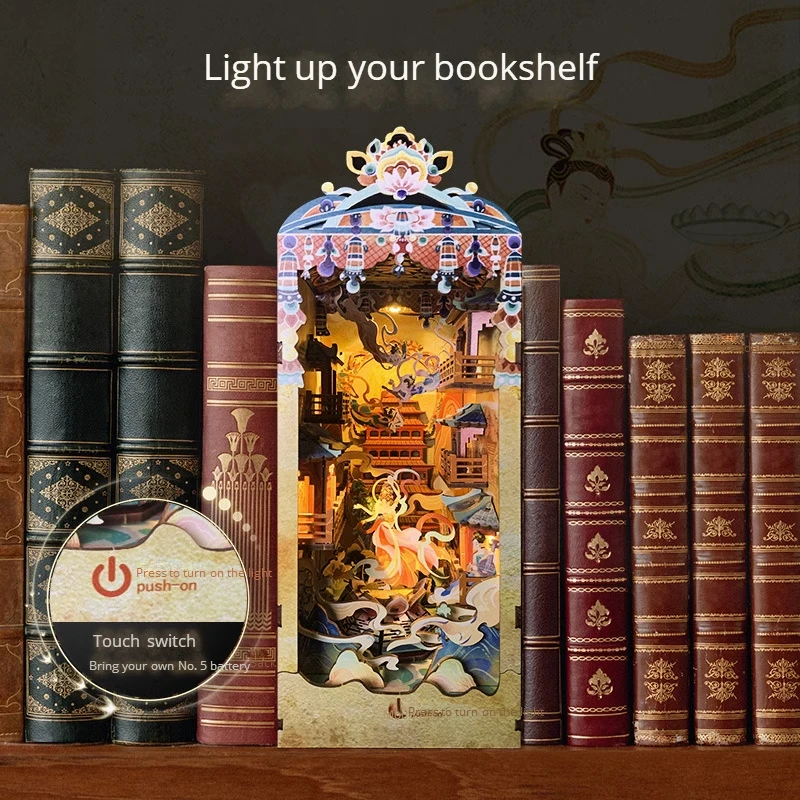The image is an advertisement showcasing a unique decorative item designed for bookshelves. The captivating background is a dark grey, contrasting against the bookshelf, which is a medium brown hue. At the top of the image, the words "Light up your bookshelf" are emblazoned in white letters, guiding the viewer's eye to the main attraction. The shelf features an array of visually striking books: on the right-hand side, three or four leather-bound volumes adorned with elaborate gold gilded patterns stand proudly; in the middle, there is an exceptionally intricate, multicolored artwork resembling a traditional Japanese or Chinese temple set amidst an architectural landscape. This central piece is not a book but a detailed 3D model that can be illuminated, creating the illusion of a miniature world nestled between the books. On the left side, two dark blue leather-bound books with silvery gilding add to the shelf's antique aesthetic. All the books appear old and important, contributing to the overall vintage charm. At the lower portion of the image, a close-up circle highlights a touch switch on the artwork, with instructions reading "press to turn on, push on, touch switch, bring your own number five battery." This detailed caption emphasizes the elegant and functional design meant to enhance any bookshelf setting.